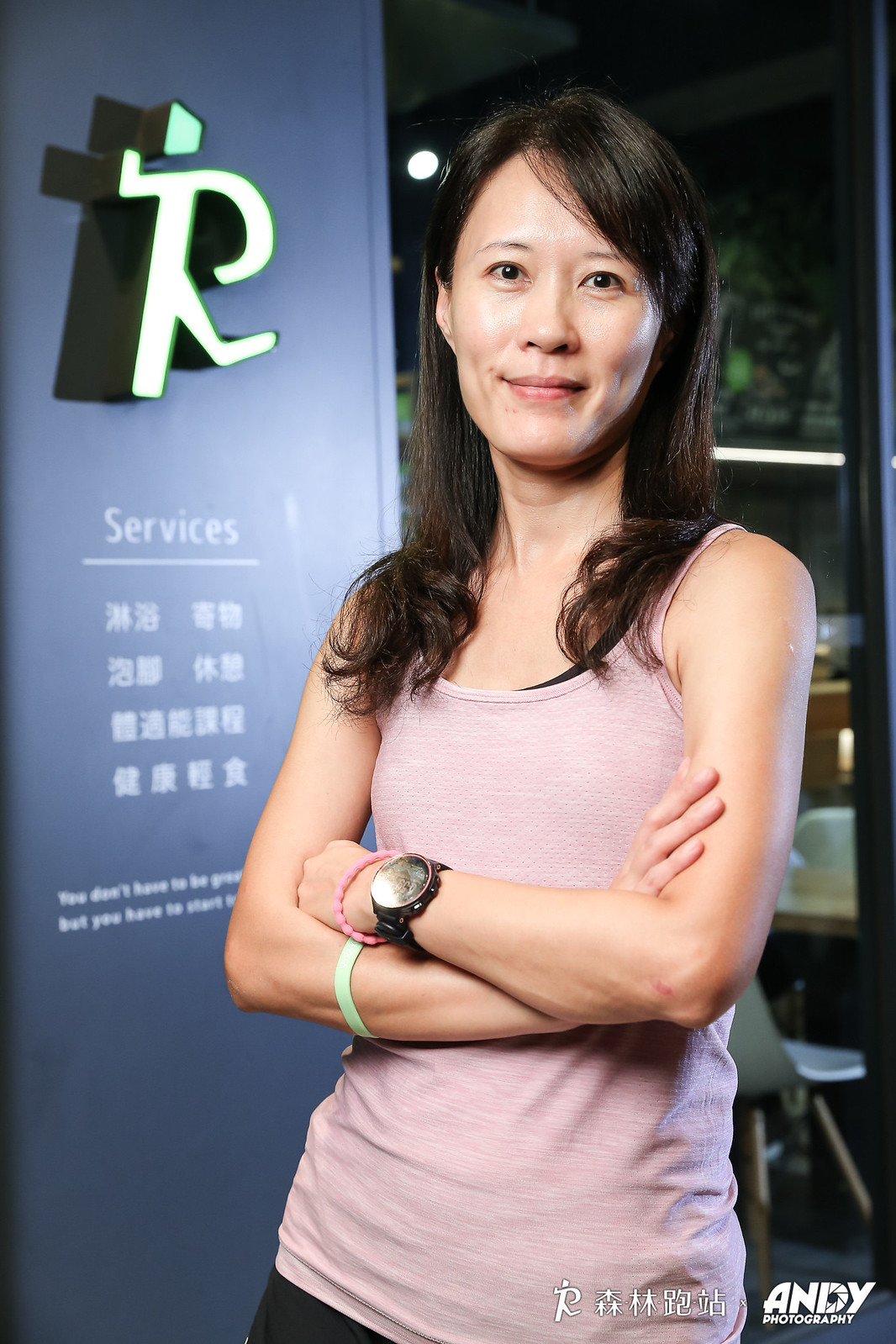The photograph features an Asian woman in her 30s standing with her arms folded across her chest. She has long, slightly frizzy black hair that extends just past her shoulders, and dark eyes. She wears a light pink tank top and accessorizes with a wristwatch and two jelly bracelets—a pink one on her left arm nearest the watch, and a light green one on her right arm. The woman gazes forward at the viewer with a slight smirk on her face.

In the background to the left, there's a sign featuring a lit-up green stick figure of a person running, accompanied by the word "services" written in Chinese characters. A chair and possibly a booth or a table are faintly visible to her right. The bottom right corner of the image contains the watermark "Andy Photography" along with additional Chinese characters.